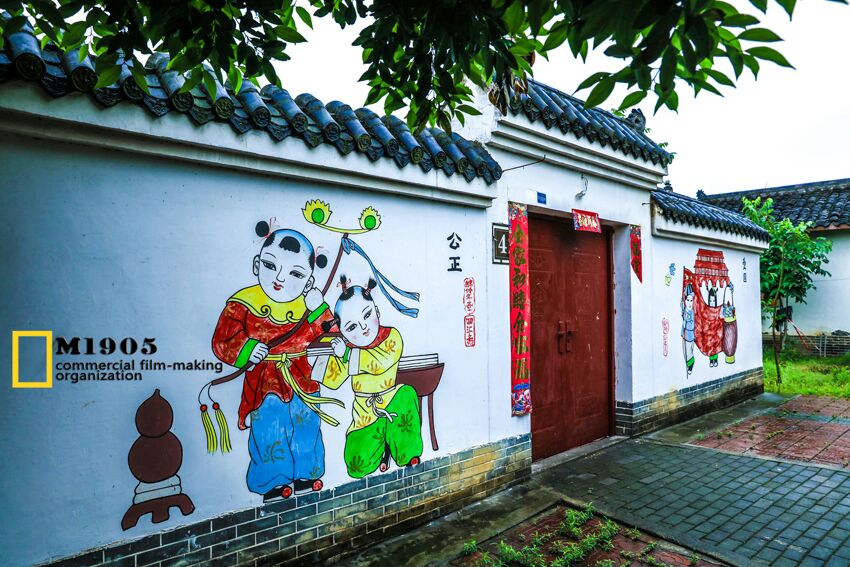This photograph captures the front facade of the M1905 Commercial Filmmaking Organization, a white building adorned with Asian-inspired elements. The building flaunts a distinctive black, clay-fashioned roof, reminiscent of the Edo period, with this roof sectioned into three parts—left, center, and right, flanked by trees. Below this striking roofline, black bricks extend up about a quarter of the way, transitioning into cyan-colored bricks on the right.

The focal point of the entryway is a pair of large red double doors, situated at the end of a black cobblestone path, which contrasts with the gray and red cobblestone surroundings. Each side of the entrance is adorned with vertical banners featuring Japanese lettering and images of children dressed in colorful, possibly traditional Japanese attire. On the left wall, two children—a girl in a red dress with blue frilled pants and a yellow-collared, holding a blue flag, and another in a yellow dress with green pants—pose close together. Another image on the right wall depicts a child in a blue dress with a matching hat and black shoes next to a peeking child behind a weaved brown basket.

Additional imagery includes a red wagon with another image of a child on the right side of the building. There’s a notable yellow sign with bold black lettering stating "M1905 Commercial Filmmaking Organization," accompanied by a white '4' within a black square near the door.

Despite an overcast sky, the building is surrounded by plentiful greenery, including grass, plants poking through the cobblestones, and trees, providing a serene yet vibrant scene reflective of both historical and cultural richness.